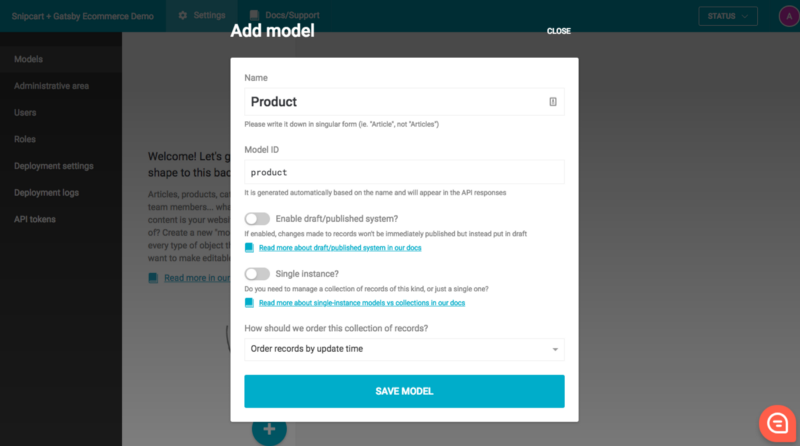The image is a screenshot from a desktop application or website, formatted for a widescreen computer monitor. The background is slightly dimmed to highlight the central pop-up box, which is the most prominent feature of the image. The pop-up, titled "Add Model," stands out against the subdued backdrop. In the upper-right corner of the pop-up, there's a "Close" button.

Within the pop-up, a white form is displayed, containing various fields and toggles for user input. The first field, labeled "Name," is intended for the user to type in the product's name. Directly below is another field labeled "Model ID," where users can enter the associated model ID. Currently, both of these fields have the placeholder text "Product."

Further down, there are two toggle switches. The first toggle, labeled "Enable Draft/Publish System," is set to off, indicated by its gray color. Beneath it is the second toggle, labeled "Single Instance?", which is also switched off and gray. 

At the bottom of the pop-up is a prominent blue button labeled "Save Model."

In the dimmer background of the image, the top left corner reveals text that reads "Snipcart and Gatsby e-commerce demo," indicating the context or platform for the screenshot.